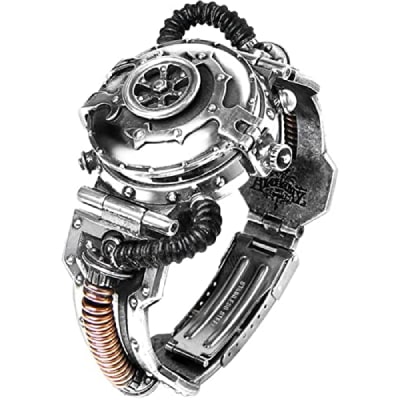This image features a detailed hand-drawn illustration of a highly intricate, steampunk-themed mechanical watch set against a white background. The watch, predominantly crafted from silvery metal, resembles a vault door with a circular, wheel-like clasp reminiscent of a submarine or even a sophisticated James Bond gadget. Notably, the watch face is concealed beneath a flip cover adorned with a metal wheel. Around the body of the device, copper-colored and black coils, as well as complex tubing, add to its industrial aesthetic. Additional etched designs embellish the wristband, hinting at the intricate craftsmanship involved. The unconventional design, complete with its elaborate metalwork and mysterious components, suggests multifunctionality beyond a typical timepiece.